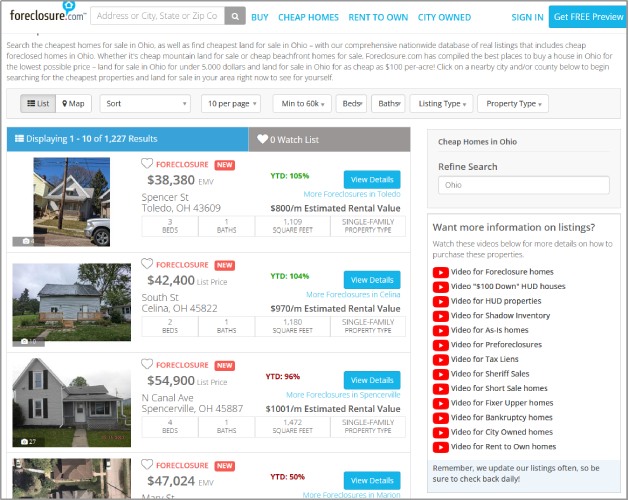The webpage features a light gray or off-white background. In the top right corner, the black text reads "foreclosure.com." Below, a search box displays the placeholder text in gray: "address or city, state, or zip, CO, then the rest of it goes north." Adjacent to this, blue text provides various options: "Buy," "Cheap Homes," "Rent to Own," "City-Owned" and "Signing." 

A blue button labeled "Get Pre-Preview" in white text appears next to a gray line extending horizontally across the page. Further down, gray text offers guidance: "Search the cheapest homes for sale in Ohio, as well as find the cheapest land for sale in Ohio." Foreclosure.com promotes its extensive nationwide database that includes rural listings, cheap foreclosure houses, and affordable land. They tout having the best locations in Ohio for purchasing houses at the lowest prices. Key listings highlighted include land for under $5,000 and properties available for $100 per acre.

The site encourages users to click on nearby cities or counties below to start searching for the cheapest properties and land for sale in their area immediately. Below this information, another section in black text reads: "List," "Map," "Sort," "Tempor," "Page," "Minimum to 260K," "Bed," "Bath," "Listed Type," and "Property Type," on a gray background.